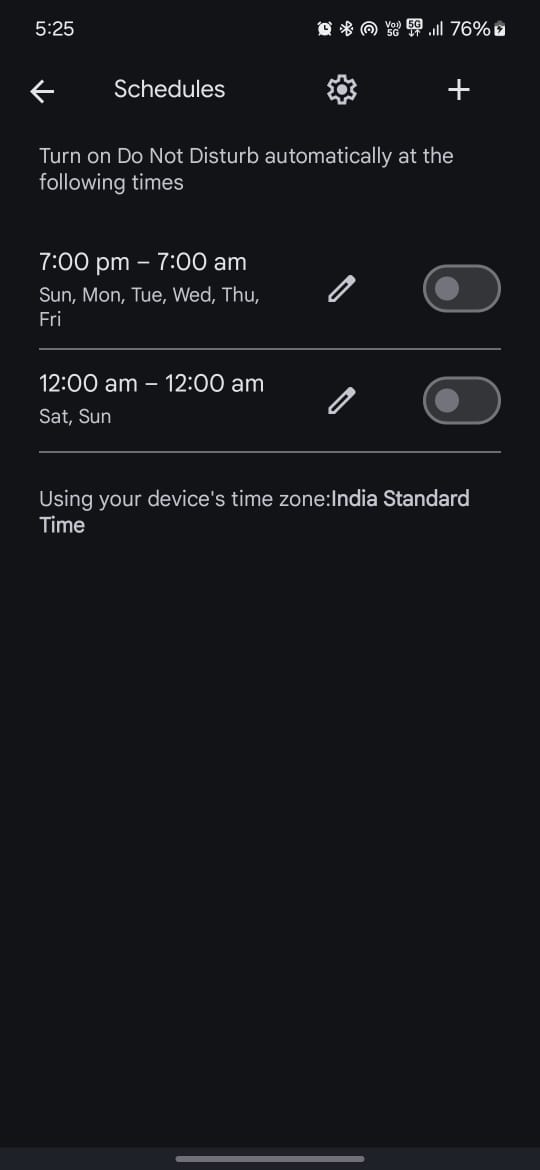The image features an application interface against a black background. At the top, the status bar displays the battery level at 76%, alongside the icons for Wi-Fi strength (5) and cellular signal (25). Below the status bar, a navigation bar includes a left arrow labeled "Schedules," a settings cogwheel icon, and a plus sign (+).

The main content area describes the "Do Not Disturb" schedules with the heading "Turn on do not disturb automatically at the following times." Two schedules are listed:

1. **7:00 PM to 7:00 AM** from Sunday to Friday.
2. **12:00 AM to 12:00 AM** on Saturday and Sunday.

Each schedule entry is accompanied by a pencil icon for editing and a gray toggle switch, indicating they are currently turned off. 

Further details include a specification at the bottom stating, "Using your device's time zone, India Standard Time," and a subtle gray line separates the content at the bottom of the screen. Overall, the interface helps users manage when "Do Not Disturb" is automatically activated.